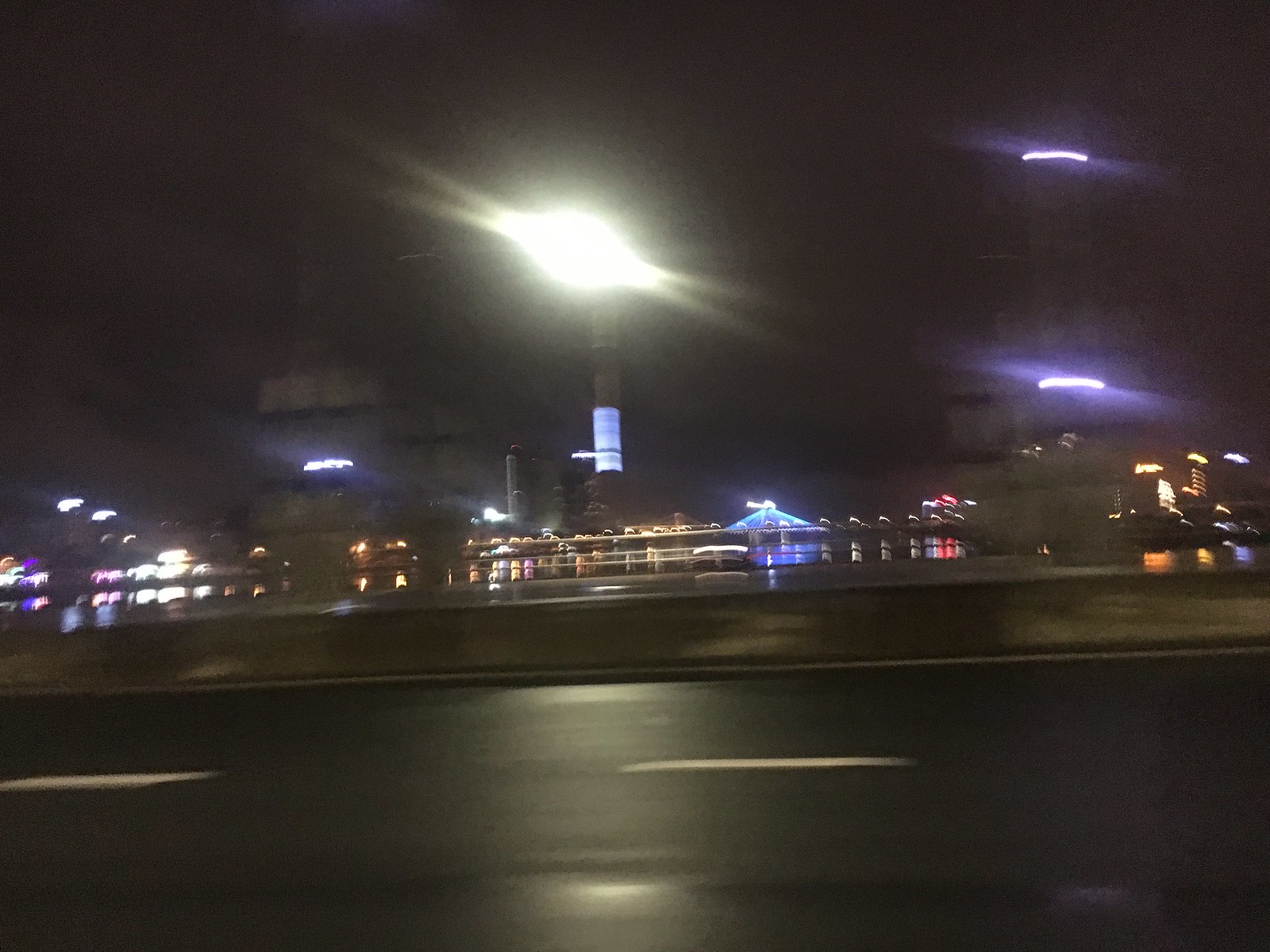This low-resolution, square-shaped image appears blurry and in motion, resulting in a fuzzy, indiscernible quality. Taken outdoors under a pitch-black night sky, the bottom portion features a dark road marked with white lines. In the background, numerous buildings, many illuminated, are visible. Among them, a prominent tower stands out, glowing brightly with white lights.